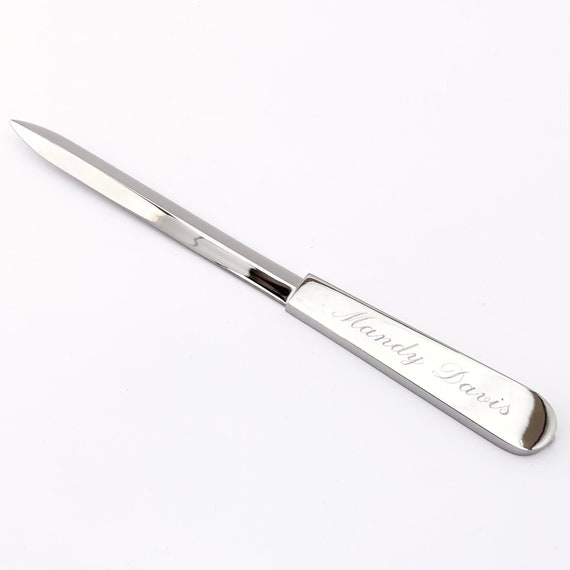The image is a detailed photograph of a silver letter opener placed on a white background, taken from a top angle in a close-up view. The object features a long, sharp, and reflective metallic blade resembling a stiletto. The handle, also made from the same reflective metallic material, displays elegant cursive text engraved in gray that reads "Mandy Davis." Both the pointed tip and the handle exhibit reflections and minor dark spots due to the lighting. There are no other elements or text present in the image.